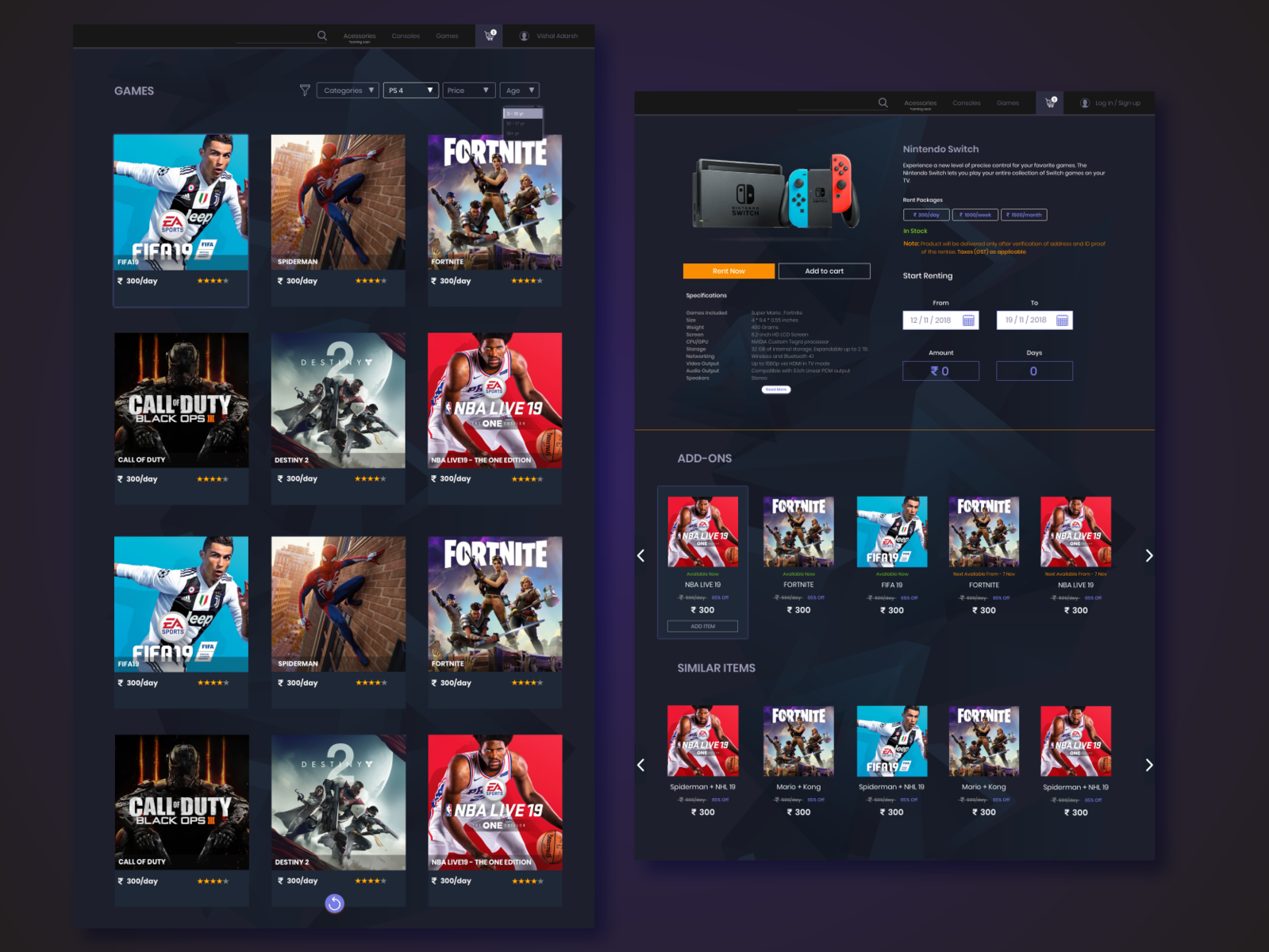The image depicts a website or an app interface, likely a launcher for video games, with a layout approximately 30% wider than it is tall. The background is a gradient of purplish-blue, lighter at the center and gradually darkening towards the edges.

On the left side of the interface, the word "GAMES" is prominently displayed in gray, all capital letters. Adjacent to this, there are four filter options—each represented by a rectangular box with a drop-down arrow—arranged horizontally. The boxes are in shades of gray and white, although the specific labels within the filters are not legible.

Beneath this section, a grid of game thumbnails is presented, laid out in three columns and four rows. Notably, the games listed repeat in sequence. The titles included in the grid are: FIFA, Spider-Man, Fortnite, Call of Duty: Black Ops, Destiny 2, and NBA Live 19. Each game appears twice in the exact order.

On the right-hand side of the interface, there's a separate section featuring an image of a Nintendo Switch. Below this image, though not entirely legible, there are areas possibly dedicated to game-related add-ons or additional content relevant to the aforementioned games on the left. The overall design is structured to provide easy navigation and access to various game options and features.